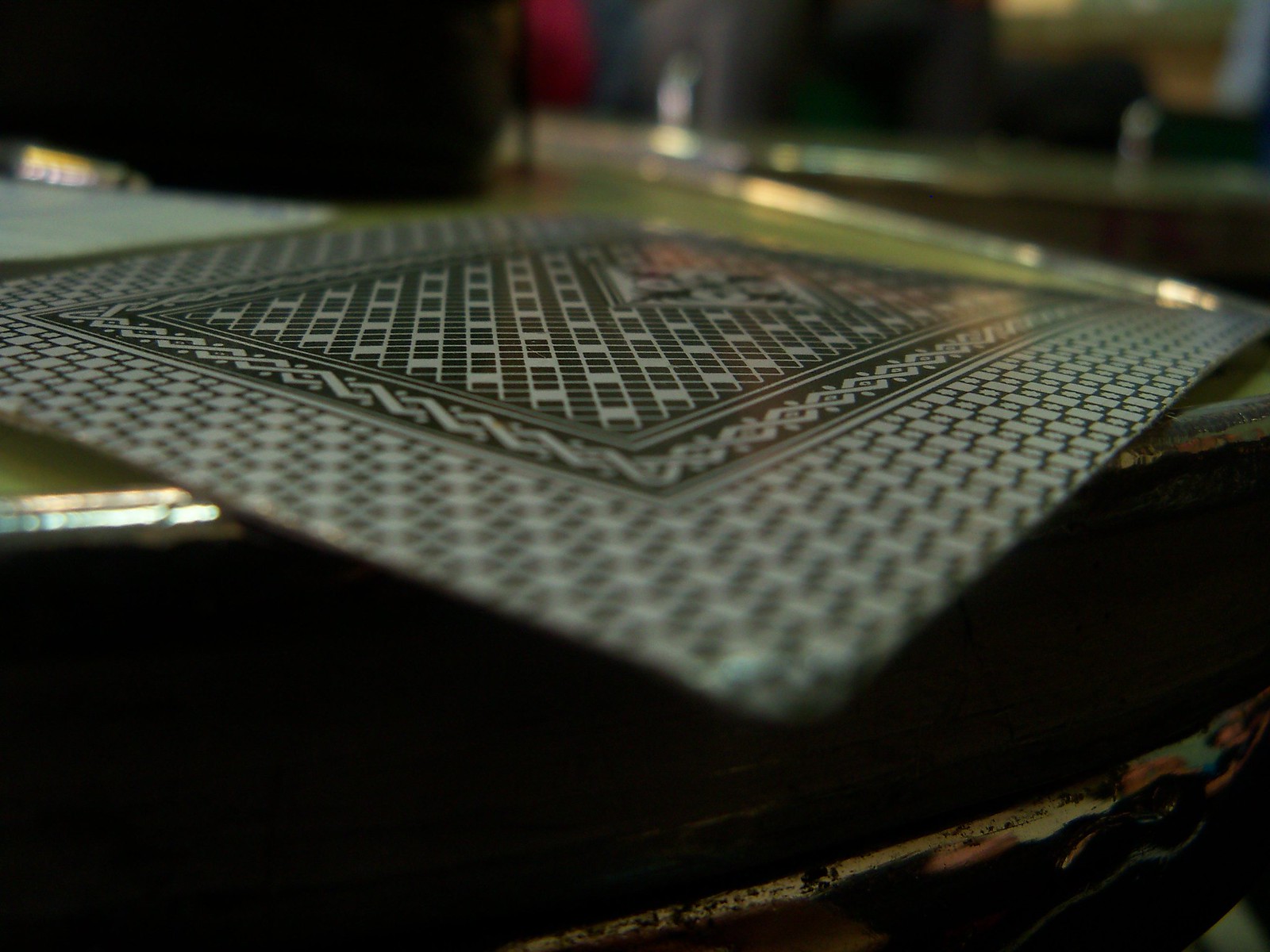This color photograph features a detailed close-up of a dark brown hardwood table edge, partially out of focus. The very bottom right corner of the image showcases a delicate enamel inset design with scalloped patterns in light pink and tan hues. The table also includes some chrome edging that is visible toward the middle of the frame. Dominating the upper half of the photograph is the corner of a playing card, adorned with an intricate black and white repeating design. The playing card displays a central square framed by a silver and black border, within which a pattern of diagonal lines creates a series of white ladder-like structures.